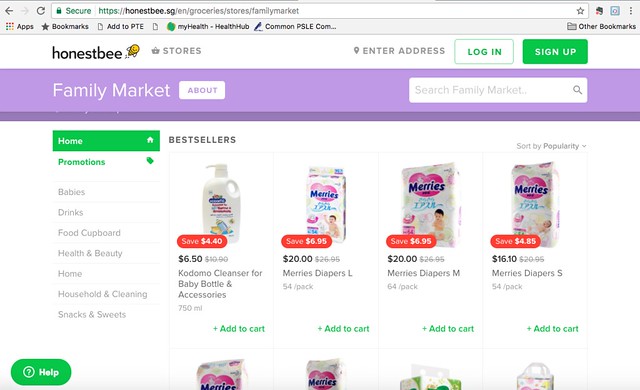A detailed screenshot of the Honest Bee website homepage is displayed. 

**Browser Navigation and Address Bar:**
- **Top Left Corner:** Displays a back arrow, a ghosted-out forward arrow, and a circular refresh icon.
- **Security Indicators:** A green padlock icon accompanied by the word "Secure" in green.
- **URL:** The address bar contains the URL "https://honestbee.sg/en/grocery/stores/family-markets" with a star icon to the far right, indicating a bookmarking option.

**Toolbar:**
- **Apps Logo:** To the left
- **Bookmark Tools:** Includes a star logo labeled "Bookmarks," a page icon labeled "Add to PTE," another page icon labeled "My Health," a pin icon labeled "Common PSLE," followed by "COM..."
- **Other Bookmarks:** A folder icon labeled "Other Bookmarks" is present at the far right.

**Website Header:**
- **Logo and Navigation:** Displays the Honest Bee logo and name ("Honest Bee"), along with a shopping cart icon and the word "Stores."
- **Location Input:** A location icon followed by "Enter address."
- **Login/Signup:** A white box with green text reading "Login" and a green box with white text reading "Sign up."

**Main Navigation Menu:**
- **Categories:** Located on the left side against a purple background, these include:
  - **Family Market Header:** The term "Family Market" is prominently displayed.
  - **Search Bar:** To the right, housing the text "Search Family Market" with a magnifying glass icon.
  - **Buttons:**
    - "About" button adjacent to the "Family Market" text.
- **Category Listings:**
  - "Home" with a green box and home icon
  - "Promotions" with a green ticket icon
  - "Babies," "Drinks," "Food Cupboard," "Health and Beauty," "Home," "Household and Cleaning," "Snacks and Sweets"
  - **Help Button:** Located at the bottom left, a blue button with a question mark icon and the word "Help."

**Main Content Area:**
- **Section Title:** Bestsellers
- **Featured Products:**
  - **Kodomo Cleanser for Baby Bottom Accessories**
  - **Mary's Diapers:** Size Large, Medium, and Small, each with an "Add to Cart" button below their respective images.
  - **Additional Products:** Partially visible at the bottom, hinting at more Mary's Diapers and other items.

This account details the layout and key elements of the Honest Bee website, providing clear navigation and product information for the online user.